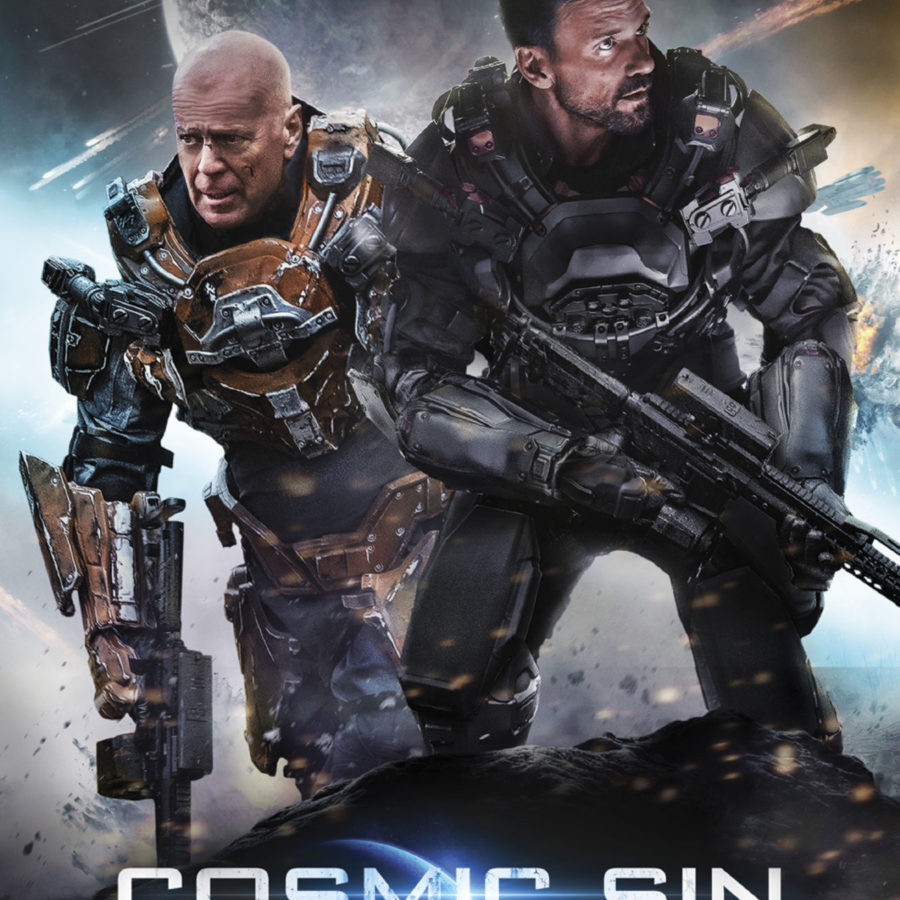The image is a full-color, sci-fi themed movie poster with the title "Cosmic Sin" partially visible at the bottom. It prominently features two heavily armored soldiers standing on a rugged, black rocky surface amidst a flurry of dust and debris. The left figure strongly resembles Bruce Willis, with a bald head and an orange chest piece on his otherwise black and brown mechanical armor. He holds a futuristic machine gun pointing downward. The right figure has short black hair, a black beard, and is clad in sleek, gray and black armor. He also holds a machine gun angled similarly downward and is looking to the right. The background showcases a celestial scene with shooting stars streaking across the sky and part of a moon or planet visible at the top center. Overall, the poster vividly sets a dynamic and intense atmosphere for the film.